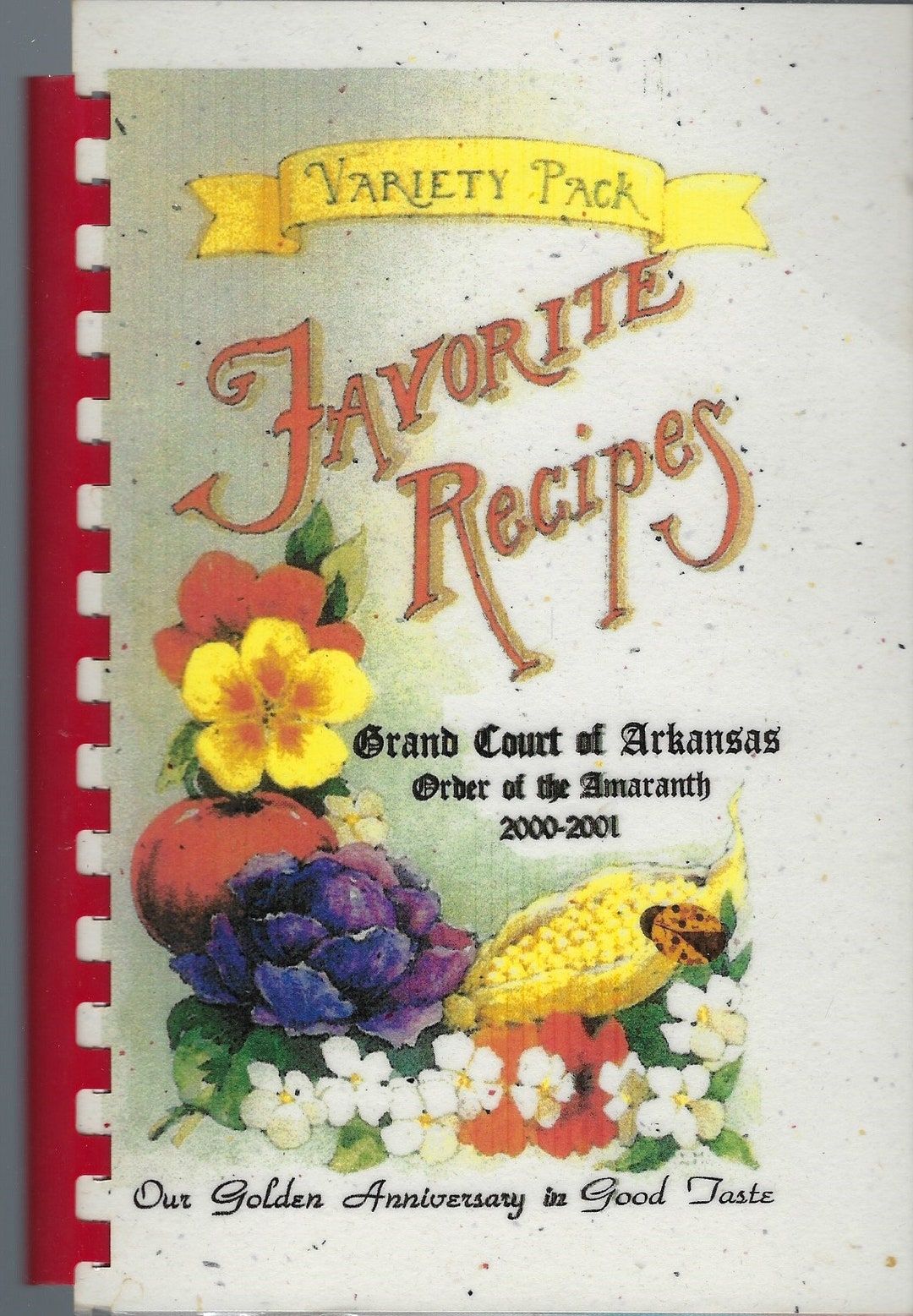This image features a colorful recipe book with a vintage charm. The book, bound together with a red plastic spiral, has white pages and a red spine. The cover is adorned with a vibrant array of flowers, including red, yellow, and white blooms with yellow centers, purple flowers, and green leaves, alongside a red tomato and yellow corn on the cob. At the very top of the cover, a yellow ribbon banner displays the words "Variety Pack." Below that, it states "Favorite Recipes" in black text, and further down, it reads "Grand Court of Arkansas, Order of the Amaranth, 2000-2001." Near the bottom, amidst more floral decorations, there's a printed message in black text that says, "Our Golden Anniversary in Good Taste." The font used throughout has a nostalgic, cursive style reminiscent of handwriting from yesteryears.